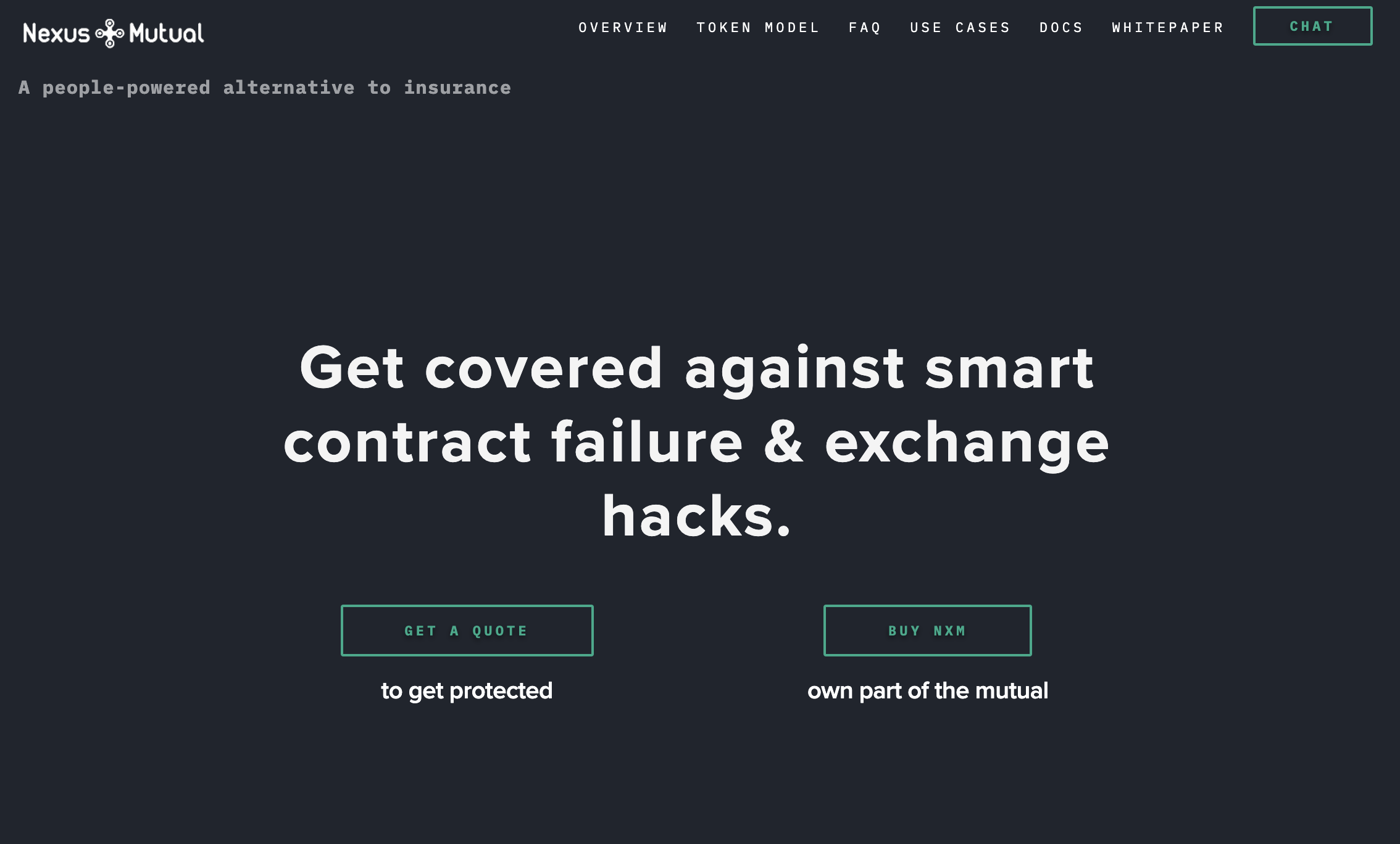Screenshot of the Nexus Mutual Website

The image showcases a screenshot of the Nexus Mutual website, characterized by its sleek black backdrop with predominantly white text. At the top, the Nexus Mutual logo is prominently displayed, featuring a unique icon resembling a plus sign with three circles at each endpoint, embedded between the words "Nexus" and "Mutual."

A horizontal menu is visible, including the following options: Overview, Token Model, FAQ, Use Cases, Docs, and White Paper. To the right of the menu, a green "Chat" button offers immediate support.

Below the menu, the tagline "A people-powered alternative to insurance" emphasizes the platform's community-driven approach. The large white text in the central area of the page states, "Get covered against smart contract failure and exchange hacks," highlighting the core services offered by Nexus Mutual.

Two green boxes are positioned beneath this headline. The first box reads "Get a Quote" with an invitation in smaller white text below, saying, "Get protected." The second box, labeled "Buy NXM," is accompanied by the message "Own part of the Mutual."

The overall layout is clean and minimalistic, drawing attention to the essential information and actions users can take. This sophisticated design aligns with Nexus Mutual’s mission to offer a modern, user-friendly alternative to traditional insurance products.